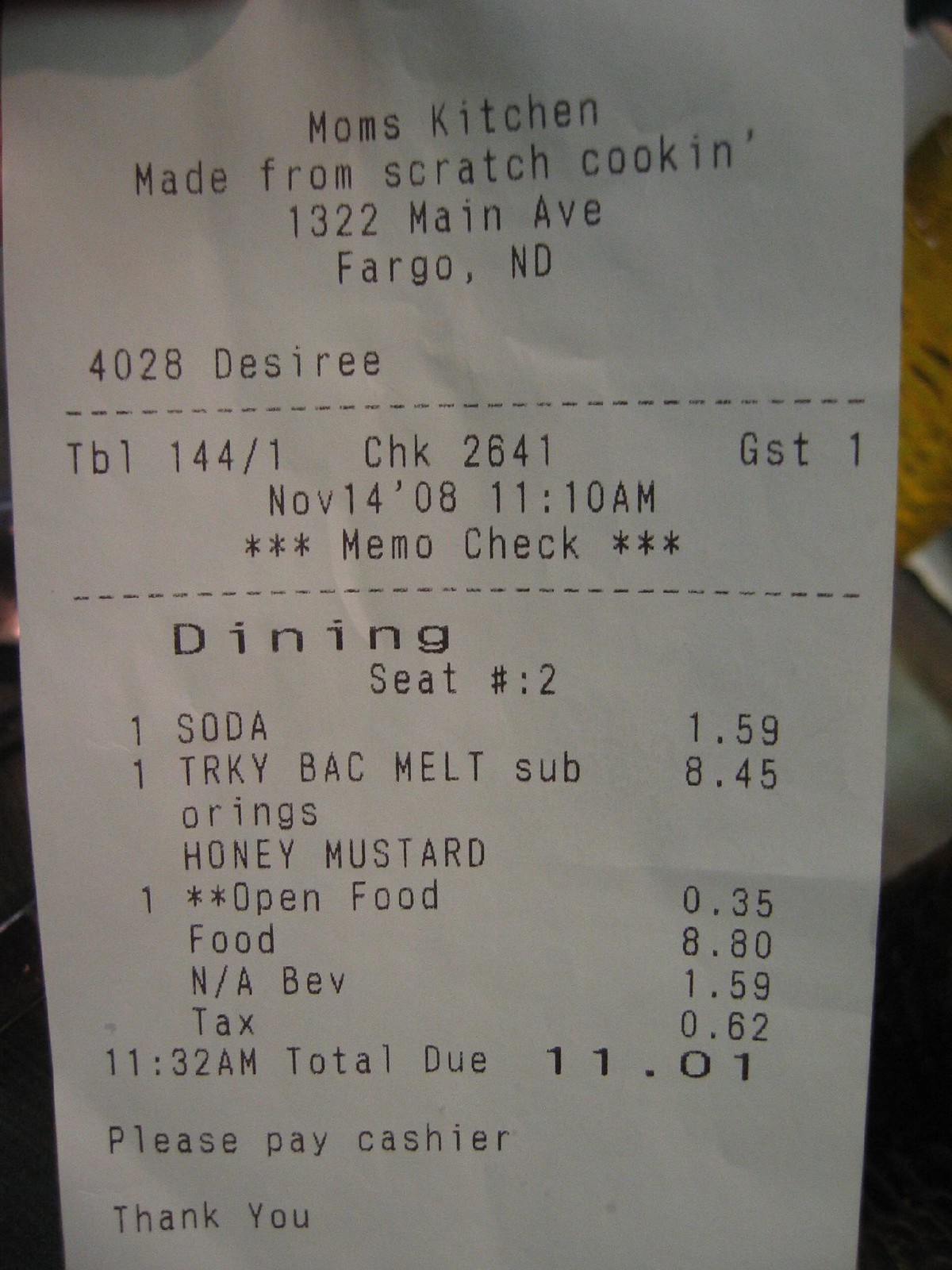This detailed image captures a photograph of a white rectangular receipt from Mom's Kitchen, a restaurant located at 1322 Main Avenue, Fargo, North Dakota. The neatly printed text at the top of the receipt confirms the restaurant's name and address. The server who attended to the guest is identified as Desiree, with some indications of table and check numbers (table 144/1, check 2641, guest 1).

Dated November 14th, 2008, the transaction occurred in the late morning, with the receipt indicating a dining time of 11:10 a.m. The specific order included: one soda priced at $1.59, a turkey bacon melt sub with onion rings and honey mustard costing $8.45, an unspecified item listed as "open food" priced at $0.35, and additional entries for food and beverage priced at $8.80 and $1.59, respectively. The receipt tallies up a tax of $0.62, bringing the total amount due to $11.01. The closing note on the receipt politely requests the guest to "please pay cashier" and extends a "thank you" at the bottom. The receipt's text is printed in black ink on a white backdrop, with minimal visible background details suggesting it was taken in a restaurant setting.